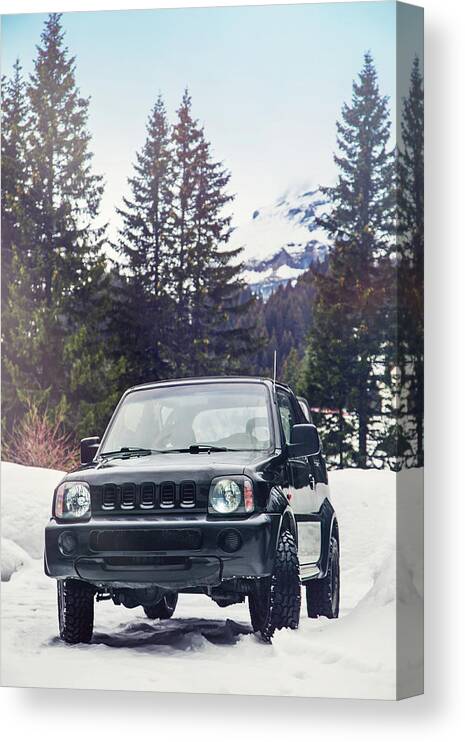The image depicts a detailed scene of a dark, black SUV, possibly a hatchback or jeep, navigating through a snowy terrain. The vehicle is positioned as if it were four-wheeling in the woods, with its tires turned to the right and snow piled up on either side. The SUV features brown headlights, a black grille, and a shadow cast below it, indicating a 3D effect. The backdrop showcases tall pine trees and a partially snow-covered mountain peak, set against a light blue, slightly overcast sky. A dead bush is visible to the left of the SUV. The entire scene appears to be part of a canvas print or box art, bringing a dynamic and immersive feel to the image.